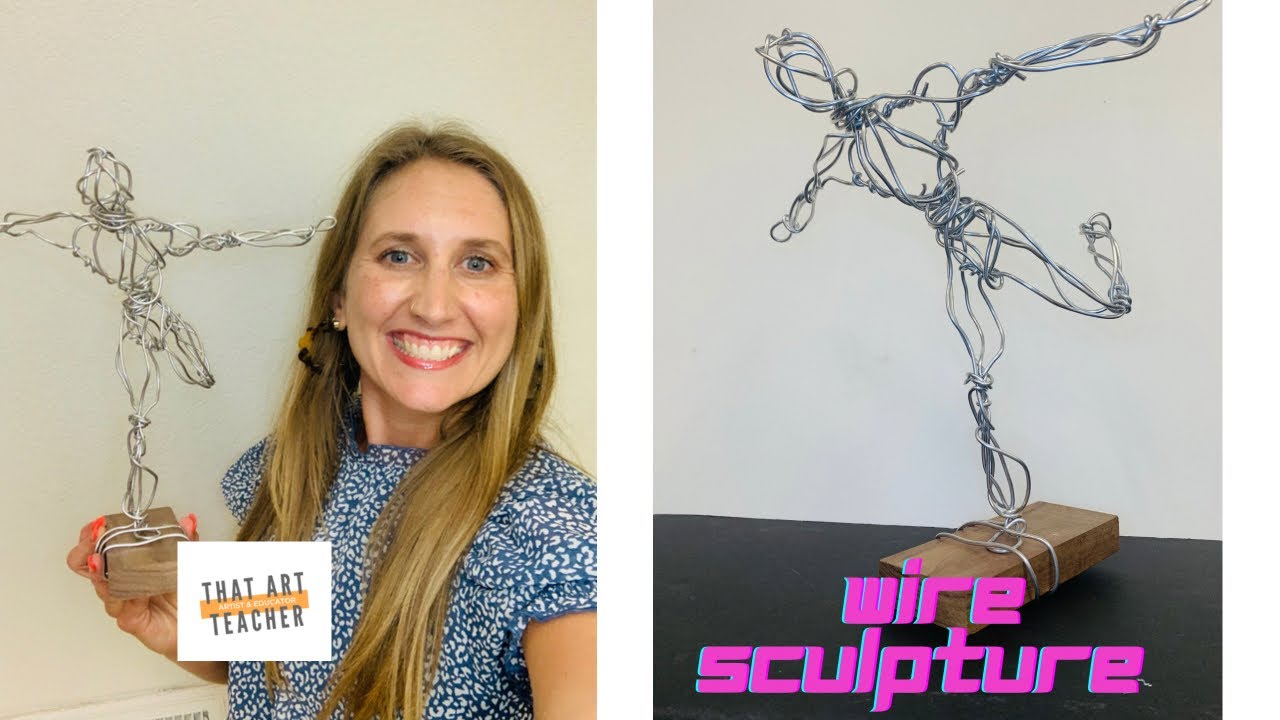The image consists of two side-by-side photos. On the left, a smiling Caucasian woman, identified by a white square caption as "that art teacher," holds a wire sculpture in her left hand. The woman, who appears to be in her early to mid-40s, has long light brown hair and is wearing a blue and white short-sleeved blouse. She sports orange nail polish and is adorned with pearl earrings. The sculpture she holds is mounted on a small wooden base, and the wire figure resembles a person with outstretched arms, one leg bent backward as if mimicking a dynamic pose or a superhero stance. 

On the right side, a close-up image of the same wire sculpture provides more detail: the figure is poised in a balancing act on the small wooden base, with wires intricately wrapped around the base to support its upright stance. This image emphasizes the sculpture's design and construction. A caption at the bottom in purple reads "wire sculpture," confirming the nature of the artwork. The background in both images is a neutral off-white, and the close-up is set against a black table, enhancing the visibility of the sculpture’s details.